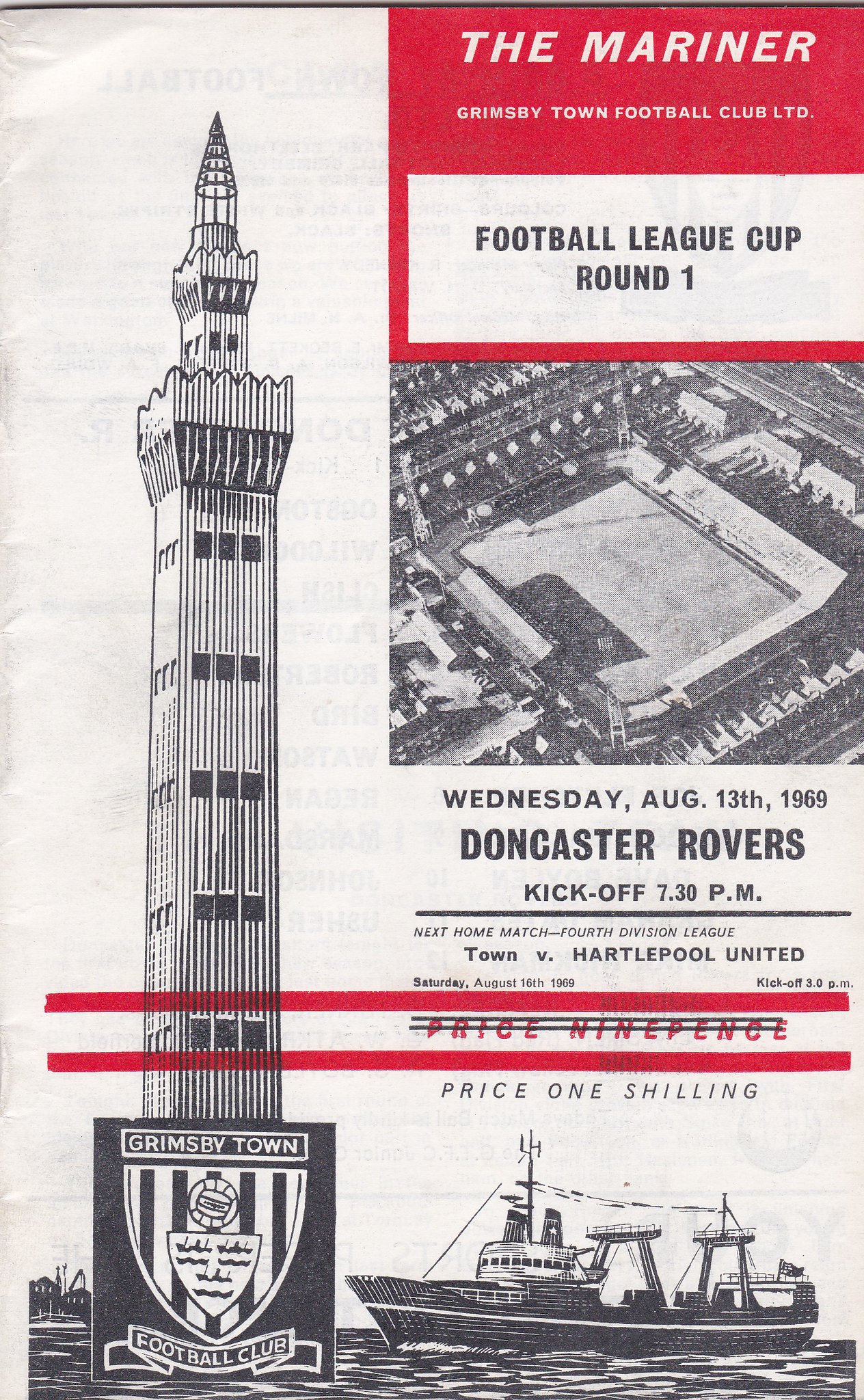The cover of this 1969 pamphlet for the Football League Cup Round 1, featuring Grimsby Town Football Club, is detailed in black and white sketch art. In the upper right corner, set against a red background, the title "The Mariner" is prominently displayed in white text. Below this title, "Grimsby Town Football Club Limited" is written, indicating the publication's association with the club. A central black and white aerial photograph showcases the Grimsby Town stadium. Also mentioned is the match detail: Doncaster Rovers vs. Hartlepool United, with the kickoff set for 7:30 PM on Wednesday, August 13th, 1969. Dominating the left side of the cover is an illustration of a tall tower appearing to rise from the ocean, alongside a small cruise ship sailing in the foreground. The tower features a sign that reads "Grimsby Town Football Club," making it a prominent emblem of the club. The overall layout of the pamphlet is visually striking, with a mixture of text and images that encapsulate the essence of this historic football event.